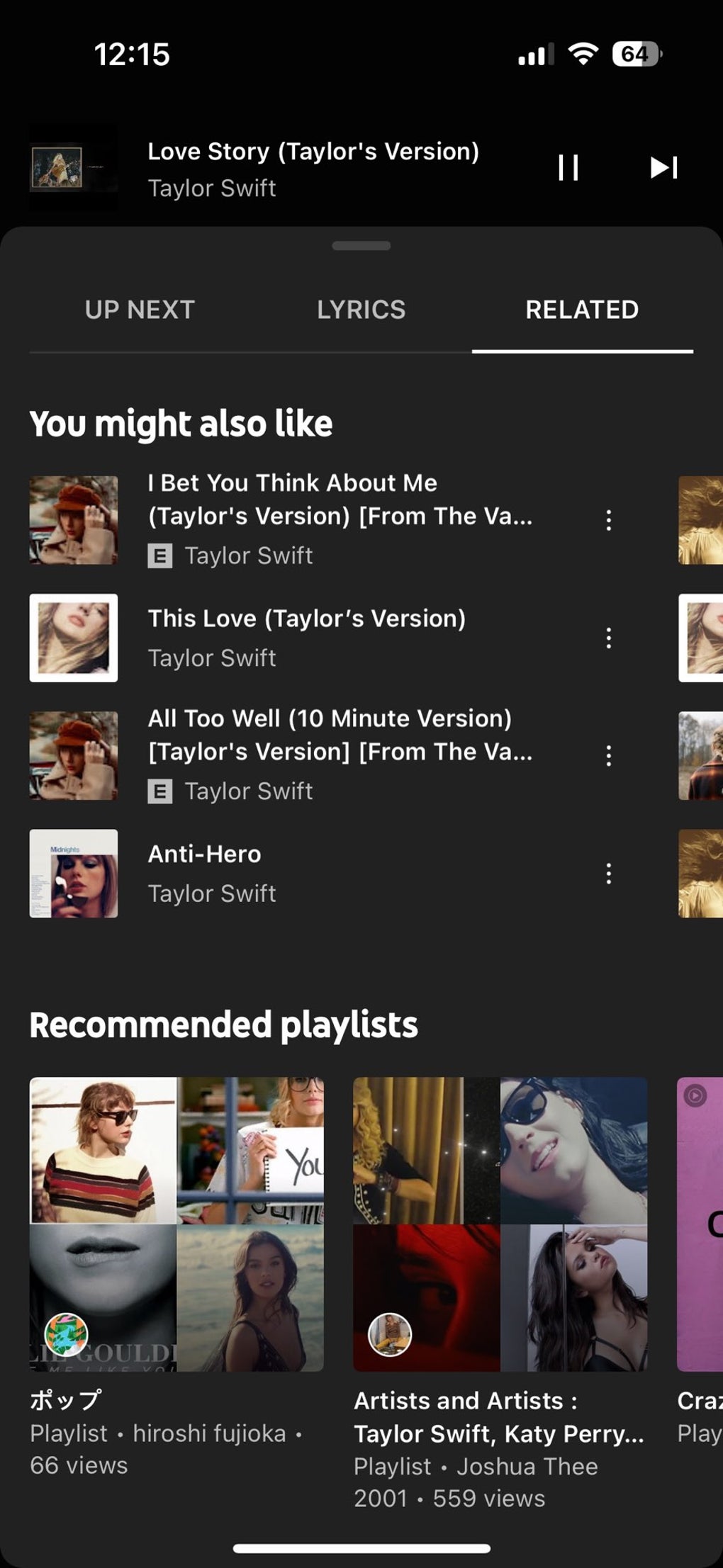The image displays a smartphone screen oriented vertically with a predominantly black background transitioning to dark gray. At the top, the background is a solid jet black, which gradually fades into dark gray below.

In the upper left-hand corner, the time is prominently displayed as "12:15," alongside the signal strength bar icon, the Wi-Fi icon, and the battery icon indicating 64% charge.

On the left-hand side of the screen, there is a small album cover with white text reading "Love Story (Taylor's Version)" by Taylor Swift. Below the album cover, there are play and pause icons.

The interface below switches to dark gray, featuring three selectable options: "Up Next," "Lyrics," and "Related," with "Related" currently highlighted and underlined.

In bold white text, the section titled "You Might Also Like" presents a series of album covers accompanied by song titles and artist names, all by Taylor Swift. The list includes:
- "I Bet You Think About Me (Taylor's Version) (From The Vault)"
- "This Love (Taylor's Version)"
- "All Too Well (10 Minute Version) (Taylor's Version)"
- "Anti-Hero"

Further down, another section labeled "Recommended Playlists" appears in bold white, offering additional album covers and related information underneath.